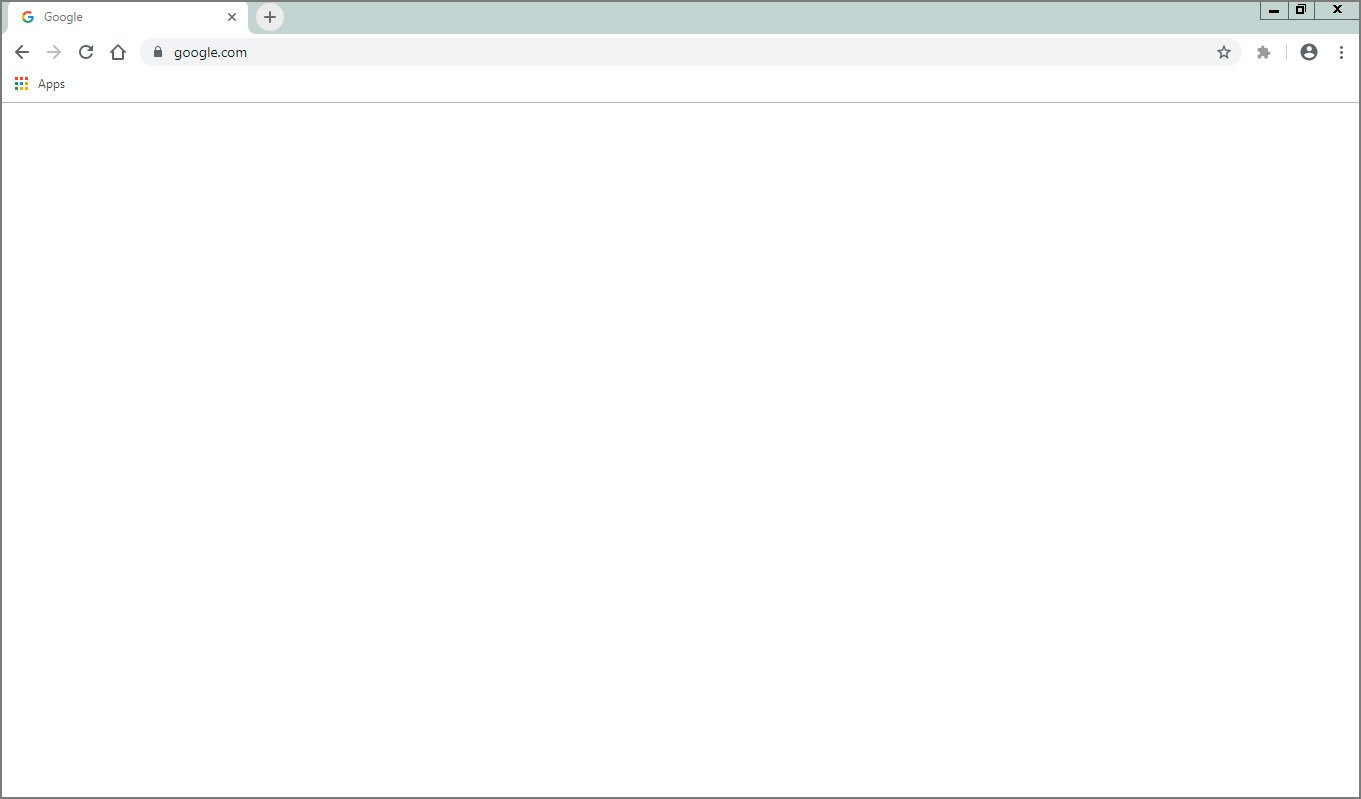A screenshot captures a minimalistic and bare browser tab open to Google's homepage. The tab, located in the upper left corner, features Google's multicolored "G" logo followed by the word "Google" in black font. An 'X' icon on the far right edge of the tab allows for closing it. Below, a light gray bar runs across the top, containing a plus sign on the left for opening new tabs and minimize, maximize, and close buttons on the right.

The browser's navigation controls are next, with a back arrow, forward arrow, refresh arrow, and a home icon aligned to the left. At the center, a search field displays "Google.com," flanked by a lock icon on the left and a five-pointed star icon on the right. Outside this search field, on the far right, are three icons: a puzzle piece, a silhouette of a person inside a black circle, and three vertical black dots for additional options.

Below this toolbar, aligned to the left, is an array of nine red dots with the word "Apps" in black font beside it, followed immediately by a thin black line. The rest of the screen is an entirely blank white page, emphasizing the minimalistic nature of the scene.